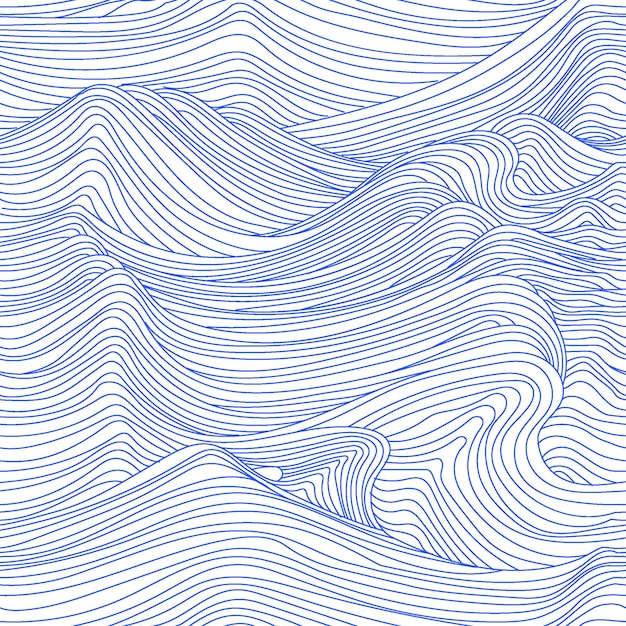The image features a detailed, abstract line drawing that predominantly resembles undulating ocean waves. Rendered in thin blue lines against a white background, the artwork uses a single line to form each wave, creating an effect that captures the natural, flowing motion of the sea. The lines are consistent in weight, and towards the right side of the image, some crests appear, reinforcing the ocean wave interpretation. While there is a suggestion that the drawing could also depict wind patterns or an aerial view of a mountain range, the fluidity and shape of the lines most convincingly emulate the essence of ocean waves.